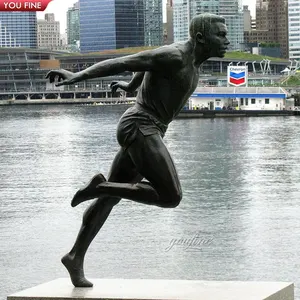The image captures an outdoor statue of a man in mid-sprint, with his right leg bent at the knee and his left foot poised on tiptoe. His arms are extended behind him, emphasizing his forward momentum. The statue, rendered in a dark grayish-black hue, stands on a white pedestal. Notably, the sculpted figure features intricate details, with what appears to be sweat dripping down his face, adding a sense of intensity and motion. The racial identity of the statue is ambiguous due to its monochromatic color.

In the background, a body of water separates the statue from a bustling downtown cityscape. Prominently visible is a small white building with blue signage that reads "Chevron," reminiscent of the gas station logo, suggesting it might serve a marine purpose. Beyond this, tall skyscrapers dominate the scene, their numerous windows reflecting the activity and vibrancy of the urban area. In the top left corner of the image, there is text that reads "YOU FINE" in white, overlaid on a red banner, adding an intriguing, possibly playful element to the composition.